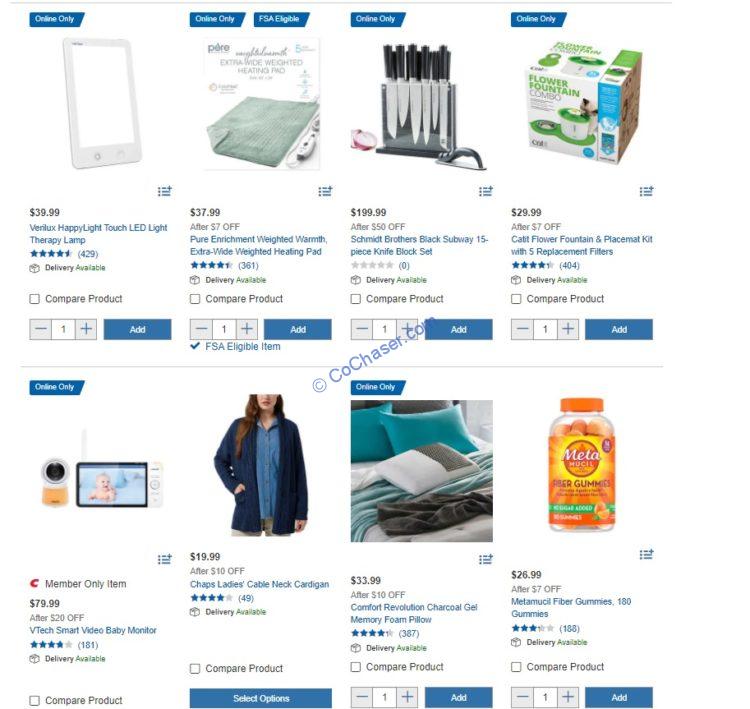The image depicts a shopping interface, capturing either a computer or mobile screen while browsing various products. Prominently featured at the top of the page is a Verilux HappyLight Touch LED Light Therapy Lamp, priced at $39.99. This item boasts a robust rating of four and a half stars based on 429 customer reviews. An online-only icon is displayed in the corner, indicating exclusive availability on the web.

Below the product name, essential details are methodically arranged: the price of the item, its rating, the number of reviews, and whether delivery is available. Users can adjust the quantity using a plus and minus control, set at a default value of one. Adjacent to this quantity selector is a blue "Add" button for adding the item to the shopping cart. Each product entry maintains a uniform layout, including a thumbnail image, price, any applicable discounts, the item's name, star rating, number of reviews in parentheses, delivery availability, a "Compare Product" option, and the quantity selector with the corresponding "Add" button.